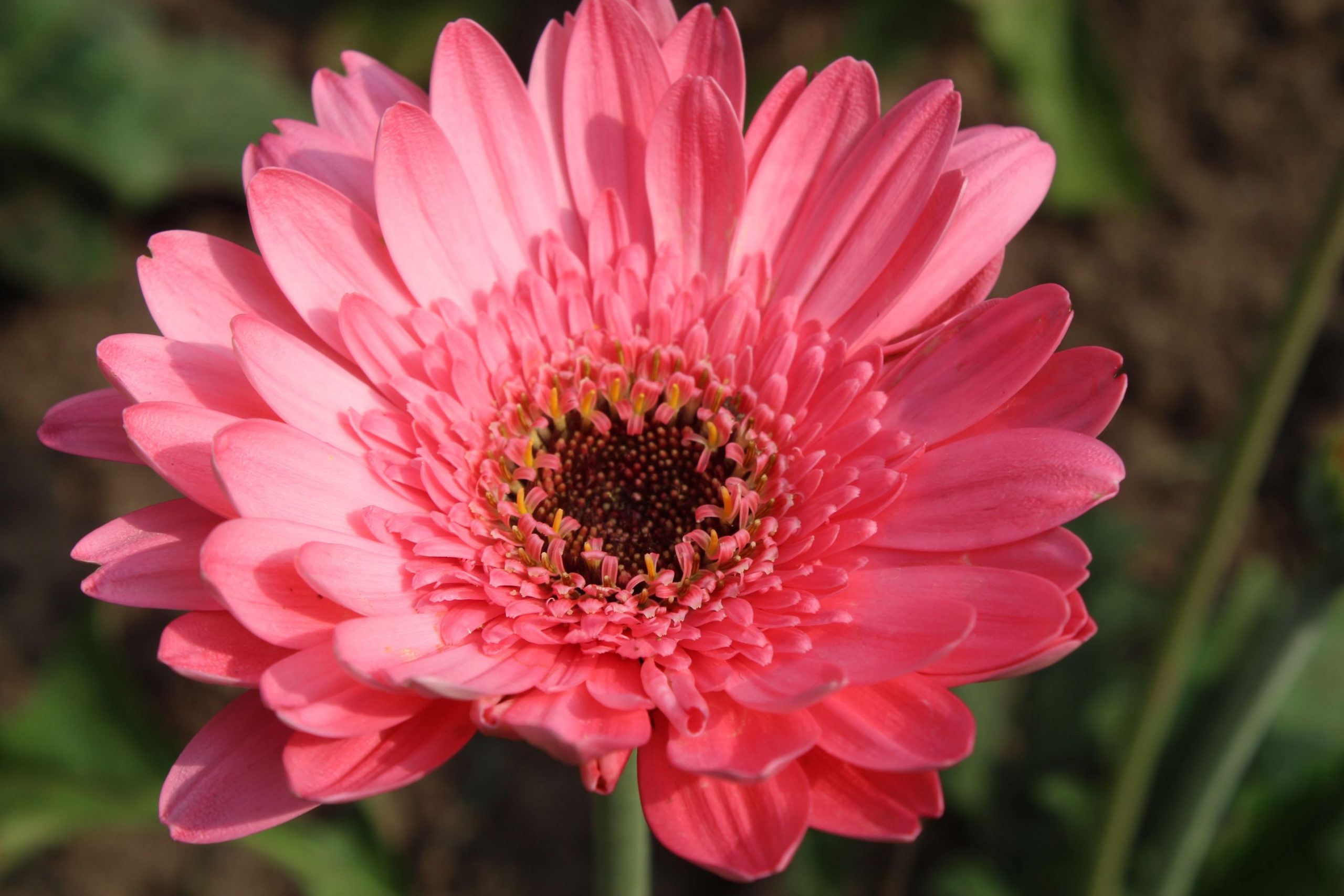This is an extremely detailed and close-up photograph of a single, vibrant pink flower. The flower features numerous layers of long, delicately lined pink petals that radiate outward, with smaller pink petals densely packed in the center. At the very heart of the flower, there is a prominent brown circular core. The pink petals appear to be finely structured, showcasing a complex, radial arrangement with at least three distinct layers and possibly over a hundred petals in total. Surrounding the flower, the background is lush and primarily green, consisting of out-of-focus vegetation, including round stems and scattered patches of dirt and leaves, particularly visible in the top right corner. The healthy green stem of the flower is slightly visible, adding to the impression of the flower being ready for pollination.